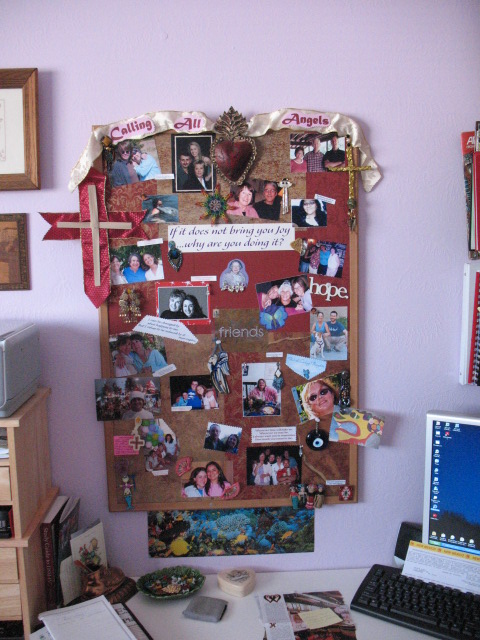The photograph depicts a detailed view of a workspace, presenting a captivating glimpse into someone's personal and creative environment. The scene is dominated by a cork board situated on a light orchid-colored wall, behind a white-top desk filled with various items. The cork board, bordered by light brown wood, is filled with a rich assortment of photos, trinkets, and inspirational words, giving it the appearance of a carefully curated montage. A prominent cream ribbon stretches across the top with the phrase "Calling All Angels" in purple text and a heart in the middle. Directly beneath this ribbon, towards the center, is another notable piece of paper reading, "If it does not bring you joy... why are you doing it?" A mix of words like "friends" and "hope" appear amidst the collage, which also features images of people, a few crosses, and numerous slips of paper. To the far right, a gray computer monitor peeks into the frame, accompanied by a black keyboard. The desk below features a green tray, books, a magazine, a small ashtray or container, and possibly a tablet, indicating an active, multifaceted use of the space. Adjacent to the cork board are wooden shelves holding what looks like a printer, and two framed photos hang above. The scene conveys a sense of personal inspiration and productivity, infused with the personality and interests of its owner.